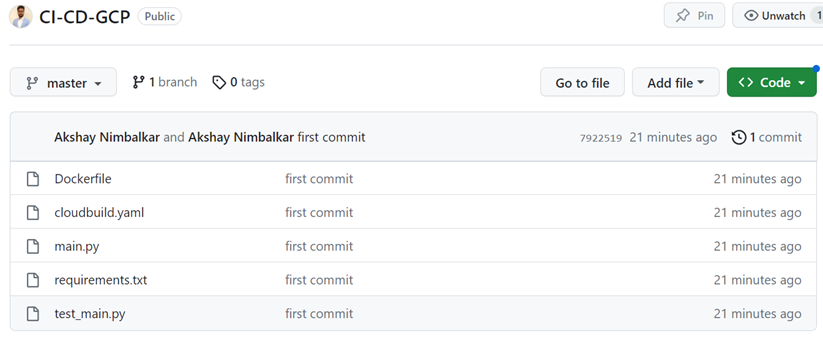This screenshot depicts a section of a version control interface, possibly GitHub. In the upper left corner, the user profile picture is visible along with labels for CI, CD, and GCP, followed by a "Public" button. On the opposite corner, there are options to pin or unmatch the repository.

Beneath the top bar, on the left side, a drop-down menu labeled "master" indicates the current branch, showing there is one branch and zero tags available. On the right-hand side, functional buttons labeled "Go to file" and "Add file" are present, each accompanied by a drop-down arrow. The interface also features a green "Code" button with a drop-down arrow.

The main content area lists several files, each with metadata indicating their status and recent activity:
1. **Akshay Nimklar**: Shows as the commit author for the first comment, timestamped 21 minutes ago, with a mention of one comment. Files include:
   - **Dockerfile**: Marked as "First commit," dated 21 minutes ago.
   - **Cloud Build YAML**: Also marked as "First commit," dated 21 minutes ago.
   - **main.py**: Labeled as "First commit," dated 21 minutes ago.
   - **requirements.txt**: Tagged as "First commit," dated 21 minutes ago.
   - **test_main.py**: Noted as "First commit," dated 21 minutes ago.

Overall, this screenshot captures the initial setup and commit details of a project repository, highlighting recent file additions and the associated author information.